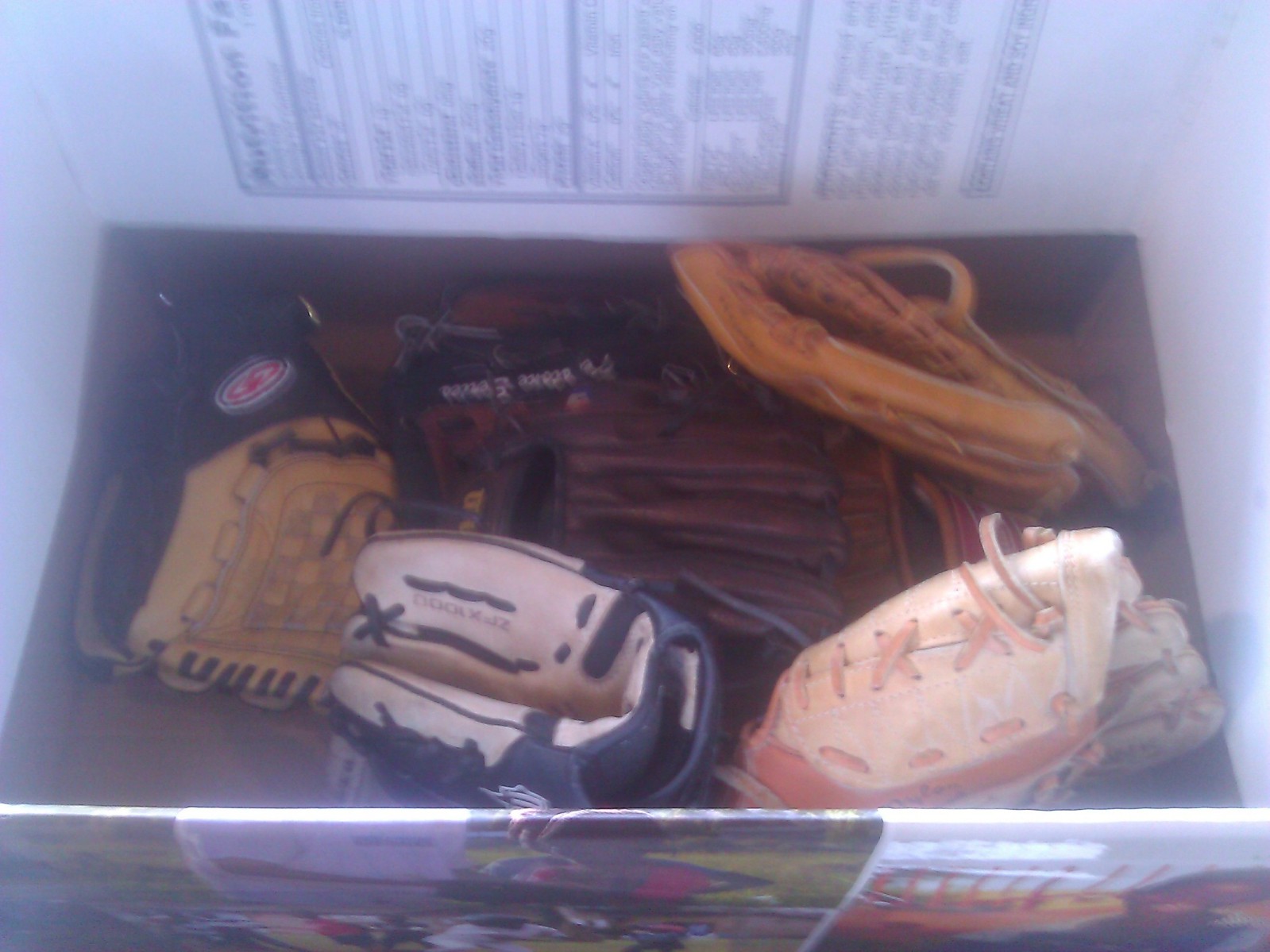The image depicts a repurposed cardboard box originally used for food, evidenced by visible nutritional facts and colorful food imagery on its sides. This box now contains a diverse assortment of baseball gloves. The gloves come in various colors and materials: a white glove with tan accents, a blue glove with tan details, a yellow glove, a dark brown glove, and another even darker brown glove. Additionally, there's mention of a yellow glove with black fringes, a white and blue glove with blue fringes, and an orange glove with pink fringes. Each glove features some form of lettering, though the image clarity prevents the text from being easily readable. The haphazard arrangement of the flaps of the box further emphasizes its secondary use, and amidst the gloves, there appears to be an indistinct image of a baseball player on the box, adding to the sporting theme.